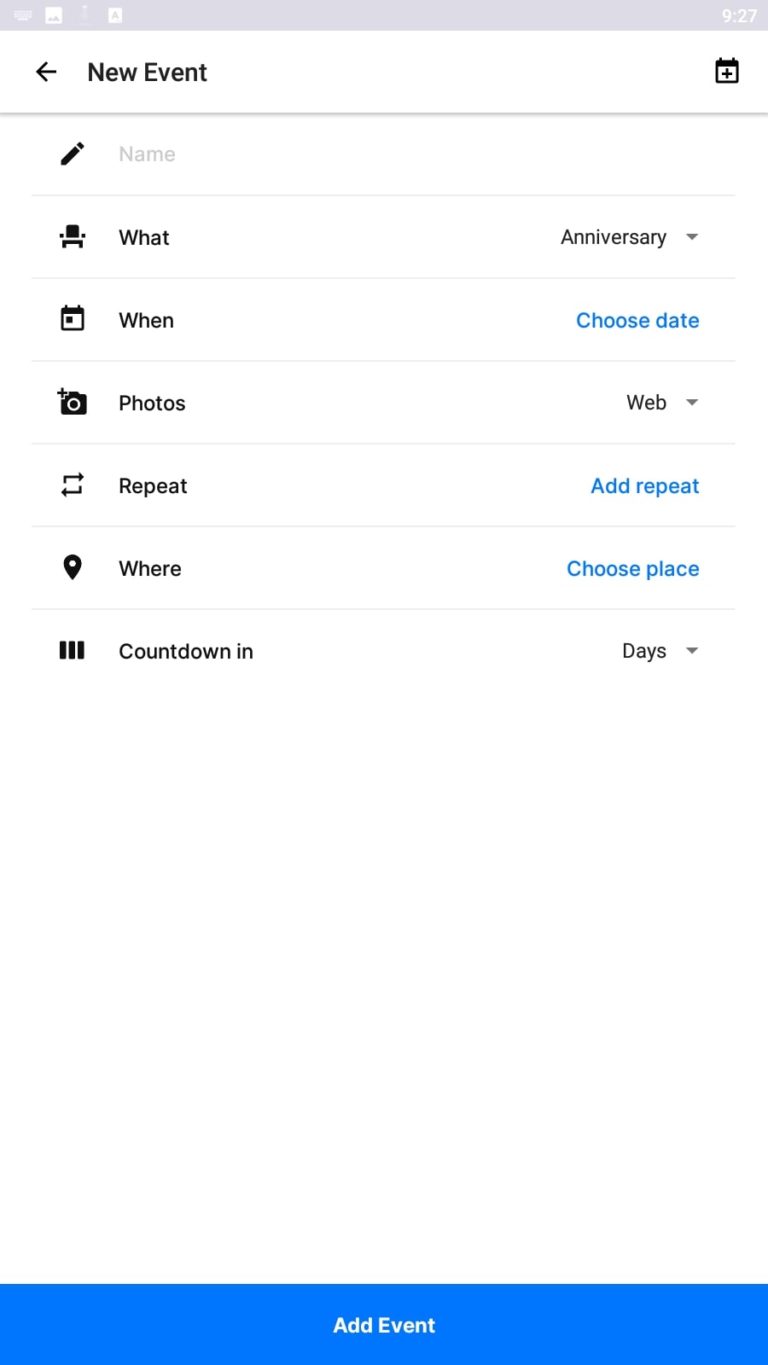This screenshot captures a mobile phone interface at 9:27 AM, as indicated by the time displayed in the upper right corner. The topmost section features a light gray bar with a partially open hamburger menu on the top left. Below this, the screen is focused on creating a new event.

On the top left, there's a back arrow for navigation, while the top right corner showcases a calendar icon with a plus symbol. Immediately below, the interface begins with a pencil icon labeled "Name" which is followed by a chair icon next to the "What" field where "Anniversary" is typed, accompanied by a drop-down arrow.

The subsequent row displays a dark black calendar icon labeled "When," alongside a blue "Choose date" option to the right. Beneath this, a camera icon precedes the "Photos" label, with "Web" written in black featuring a drop-down menu.

Continuing down, there's a row with arrow icons pointing both left and right arranged in a square, labeled "Repeat." Adjacent to this is a blue "Add repeat" option. Further down, a pinpoint icon next to the word "Where" is positioned, with a "Choose place" option in blue on its right.

The final row before the action button features three vertical rectangular blocks in black labeled "Countdown in," beside which "Days" is mentioned in black with an accompanying drop-down menu.

At the bottom of the screen, a prominent blue button invites users to "Add event."